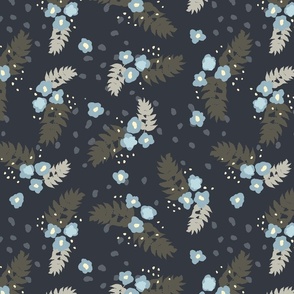This image depicts a square piece of fabric, potentially a fat quarter, featuring a winter-themed pattern on a black background. The design is characterized by dispersed clusters of light blue flowers, each adorned with a white dot at their center. Surrounding these floral motifs are delicate, feather-like leaves in shades of light tan and dirty brown, alongside dark olive green fern-like leaves. Speckled across the background are tiny white dots reminiscent of snow, interspersed with larger dark gray dots that contribute to a wintry aesthetic. The intricate pattern is evenly distributed throughout the entire square, creating a cohesive and visually appealing design. Notably, there are no watermarks, labels, or artist information present on the image.